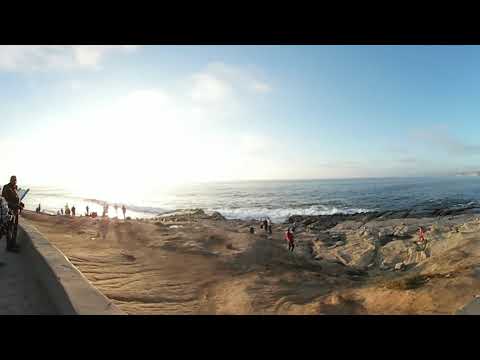This panoramic seaside image, albeit with some distortion and pixelation, captures a vibrant beach scene. The viewpoint is from a cement or concrete footpath or bike path adjacent to the beach, possibly reminiscent of southern California beaches. On this path, there is at least one person visible, seemingly looking towards us. The beach below shows signs of erosion with sandy areas intersected by rocky patches, particularly pronounced on the right side where numerous people are climbing or walking on the rocks. Further left on the smoother sandy expanses, more groups of people are scattered, perhaps some are fishing given their stance. The ocean waves, with noticeable white caps, roll energetically toward the shore under a vast, bright blue sky dotted with a few clouds. The sun, positioned mid-lower left, illuminates the scene with a brilliant white-yellow glow, enhancing the serene yet dynamic beauty of the coastal landscape.